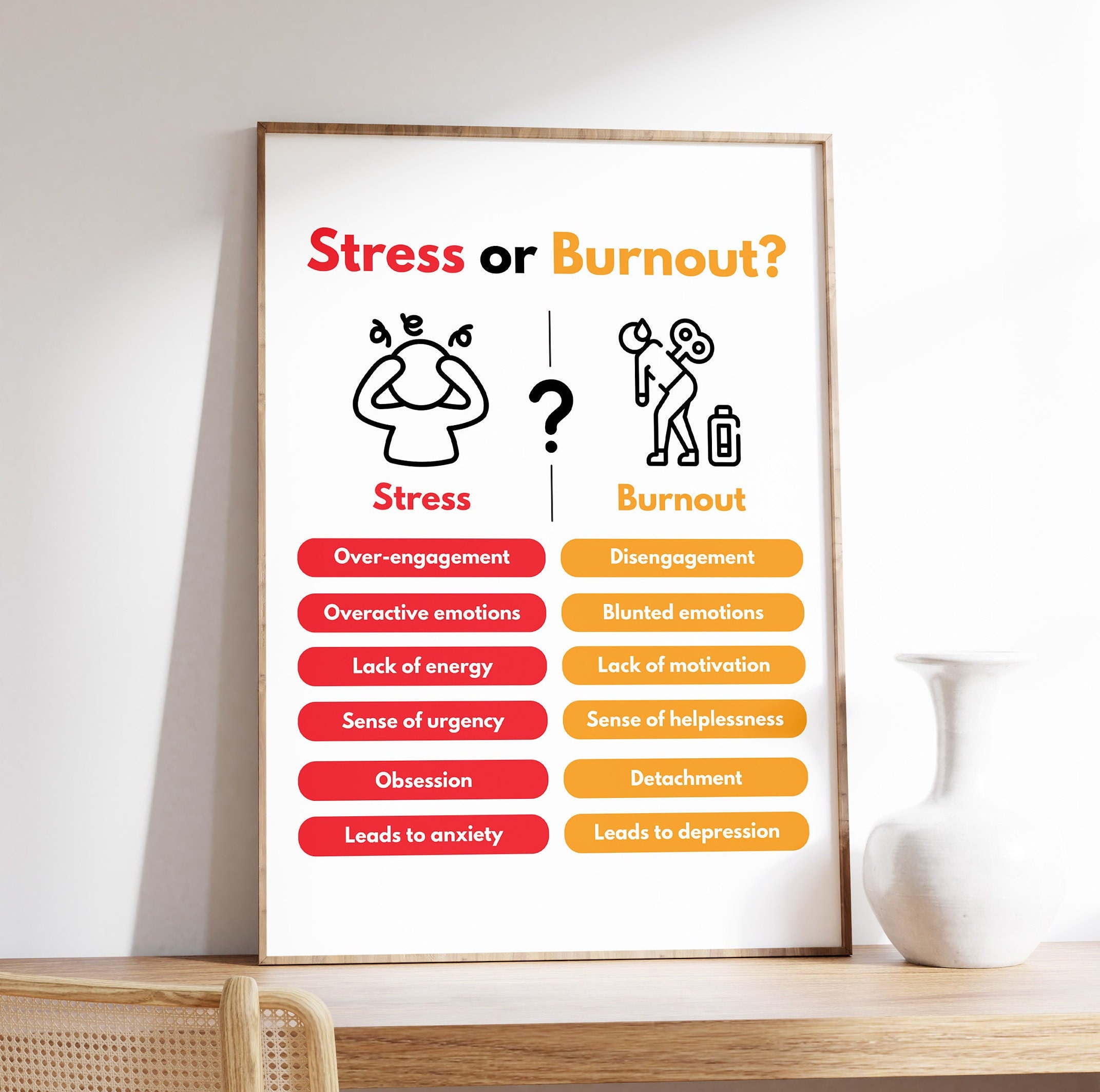The image is a large square photograph showcasing a minimalist setup against a white wall. In the center, a framed poster leans against the wall, casting soft shadows. The frame is light wood-colored, complementing the light brown wooden surface it rests on, which could be either a table or a desk. To the right of the poster sits a clean, white ceramic vase, empty and elegant. On the lower left corner, the top part of a vented wooden chair is partially visible, adding a touch of rustic charm.

The poster is divided into two sections, contrasting "Stress" and "Burnout". The title "Stress or Burnout?" is prominently displayed at the top, with "Stress" in bold black and "Burnout" in a striking orange color. Below this title, the left section displays an illustration of a person outlined in black, touching their forehead in a stressed gesture, labeled “Stress” in red. The right section shows a wind-up doll with a key in its back, symbolizing burnout, labeled “Burnout” in orange.

Under each illustration are six ovals containing characteristics associated with either stress or burnout. The stress-related symptoms, in red ovals, include overengagement, overactive emotions, lack of energy, sense of urgency, obsession, and anxiety. Meanwhile, the burnout-related symptoms, in orange ovals, list disengagement, blunted emotions, lack of motivation, sense of helplessness, detachment, and depression.

The poster serves as a useful chart for comparing the symptoms of stress and burnout, helping viewers identify whether they might be experiencing signs of one or the other.